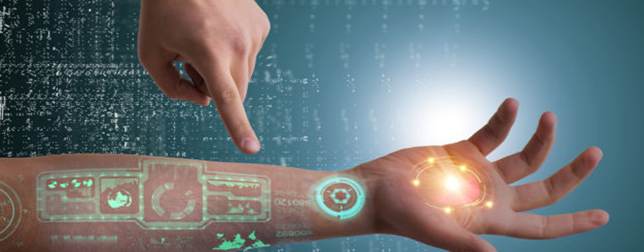The photograph showcases the right hand and forearm of what appears to be a human with a futuristic, possibly robotic, augmentation. The arm is positioned palm-up, revealing a complex holographic display over the skin. On the palm, there is a prominent yellow circle surrounded by five smaller lights or focal points. Along the wrist and extending to the forearm, a blue circular hologram with intricate gears and etched numbers is visible. This wrist section is decorated with unique patterns, adding to the technological aesthetic. The left hand is seen pointing at the holographic elements on the forearm and wrist, emphasizing these features. The background is filled with scrolling vertical lines and dots in blue and aqua hues, adding a digital, matrix-like ambiance to the scene. A bright white light underscores the futuristic theme of the image.